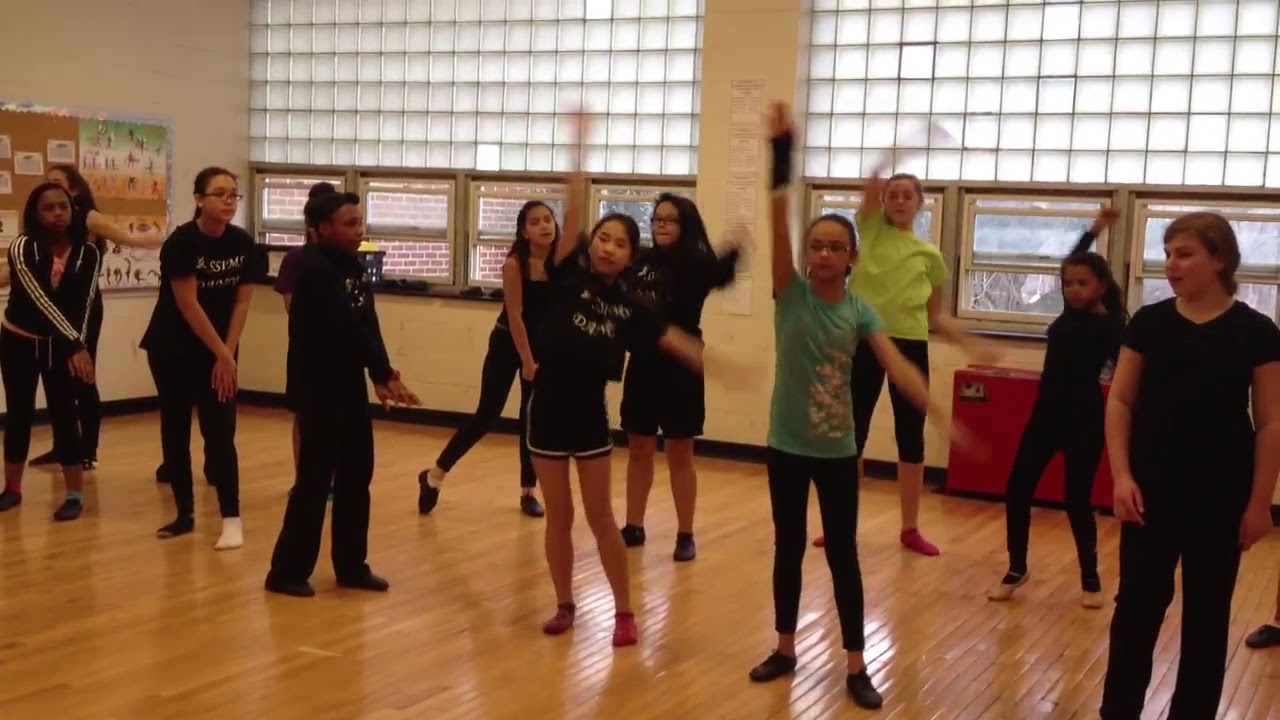The image features a class of approximately a dozen young females, likely teenagers, positioned in two rows within a spacious room with a wooden plank floor. Clustered around a wall of windows, some opaque with glass blocks above and transparent ones below, the room is bathed in natural light. The windows reveal an external red brick building and a few bushes. The group, mostly clad in black attire including long pants, shorts, and T-shirts, appear to be engaging in a yoga or aerobic session. Their poses, resembling yoga or dance movements, have them raising their right arms in a coordinated yet unsynchronized manner. A bulletin board adorned with posters is visible on the left side of the room, and nearby sits a red object, possibly an old radiator or an AC unit.